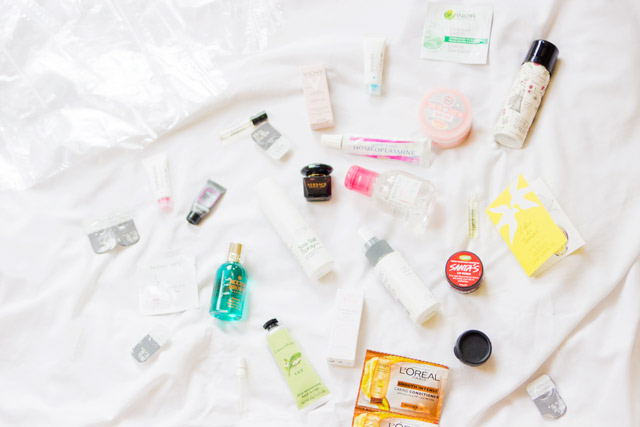This horizontal image showcases an array of beauty products meticulously arranged across a piece of white fabric, which is artfully draped with soft folds and wrinkles. The assortment encompasses a variety of packaging types and forms, from plastic and small glass jars with caps to sleek aluminum or foil packets. Highlighted among the collection are several cylindrical bottles, each featuring black caps, and one particularly striking bottle featuring a blue liquid capped with gold. Additionally, there are squeeze tubes adorned with green labels and black caps. Noteworthy items include an orange and yellow product labeled "L'Oreal" and a nearby small, circular black object. In total, approximately 18 items are scattered in different orientations across the fabric, creating a visually rich and diverse display of beauty essentials.